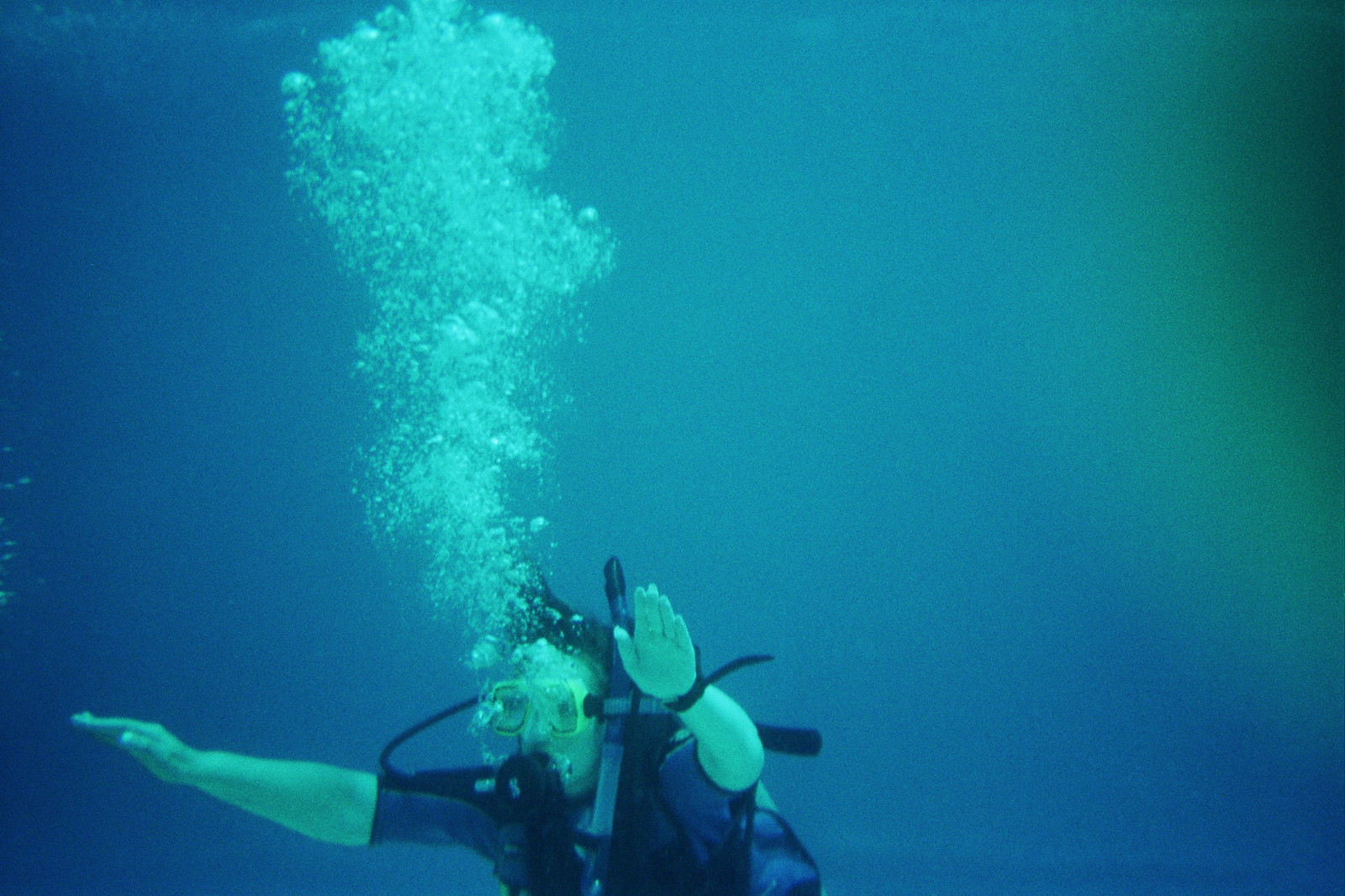In this detailed underwater scene, a scuba diver, clad in a short-sleeve, navy blue scuba suit with black straps, is captured mid-exhale, producing a massive cloud of bubbles rising towards the top of the image. The diver's arms extend outwards from his body with palms down and fingers together, akin to directing traffic underwater. His yellowish-green goggles, secured by a black band, obscure his face while enhancing the clarity of his vision in the blue, gradient water that shifts to black in the top right corner, perhaps due to a spotlight. A blue air tank strapped to his back connects to a black breather, and a black swim watch adorns his wrist. The scene is devoid of marine life, except for a slight blurry blob in the upper right that could be the photographer's finger. The diver's tense expression adds a sense of stress amidst the serene blue backdrop. The cap tightly fitted over his head is also black, completing his gear.